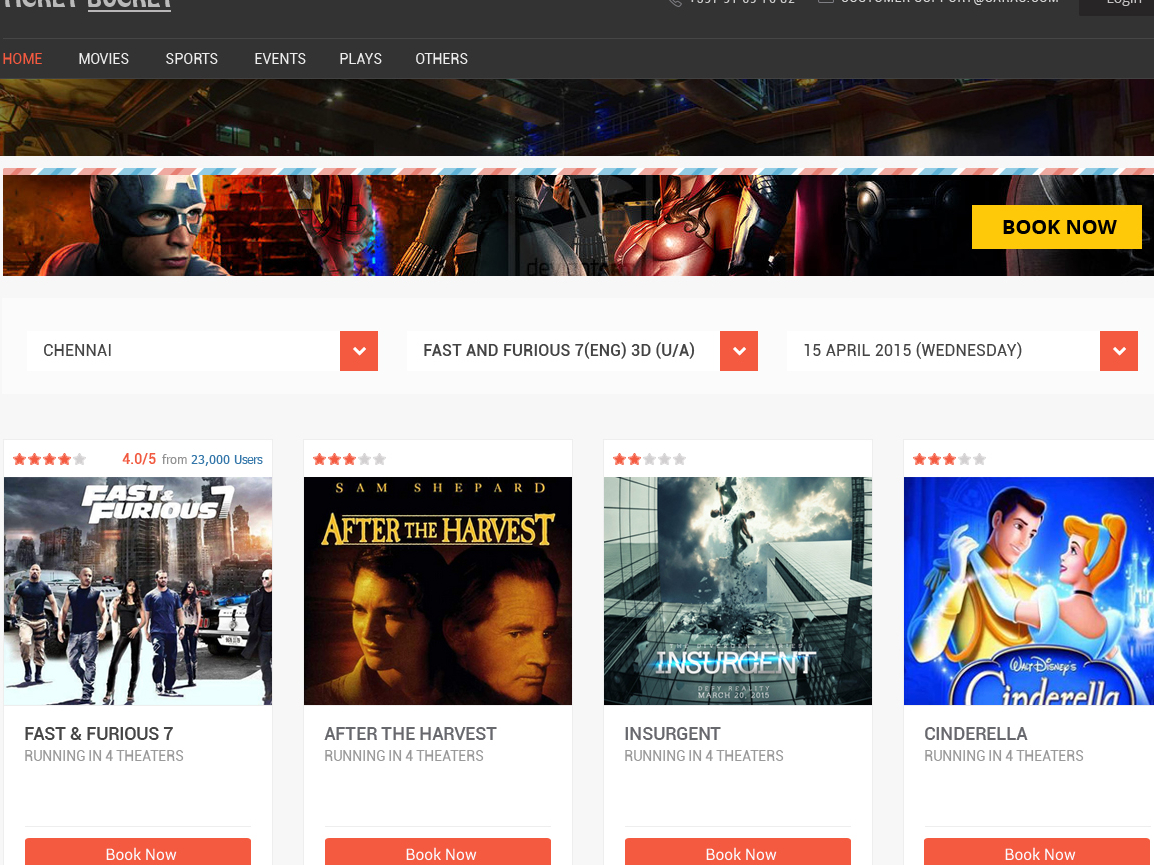This web page features a sleek black design, specifically designed for browsing films. At the top, enclosed within a black border, there are four navigational tabs: Home (where the user currently is), Movies, Sports Events, Plays, and Others. Just below these tabs, there are visuals of characters and scenes from various films, adding a dynamic touch to the interface. A prominent yellow button, captioned "Book Now" in black text, invites users to proceed with bookings.

Further down, three dropdown sections enable users to refine their choices: the first box marked “Chennai” indicates the location, the second pertains to the movie “Fast and Furious 7 (English 3D, U/A),” and the third allows users to select the date, "15 April 2015, Wednesday."

The page features four highlighted movies:

1. **Fast and Furious 7**:
   - Running in four theaters
   - Rated: 4.5 stars out of 5
   - Option: Book it now

2. **After the Harvest**:
   - Running in four theaters
   - Rated: 3 stars out of 5
   - Option: Book it now

3. **Insurgent**:
   - Running in four theaters
   - Rated: 2 stars out of 5
   - Option: Book it now

4. **Walt Disney's Cinderella**:
   - Running in four theaters
   - Rated: 3 stars out of 5
   - Option: Book it now

Each movie is represented by its official poster, adding visual appeal and aiding users in selecting their desired film effortlessly.